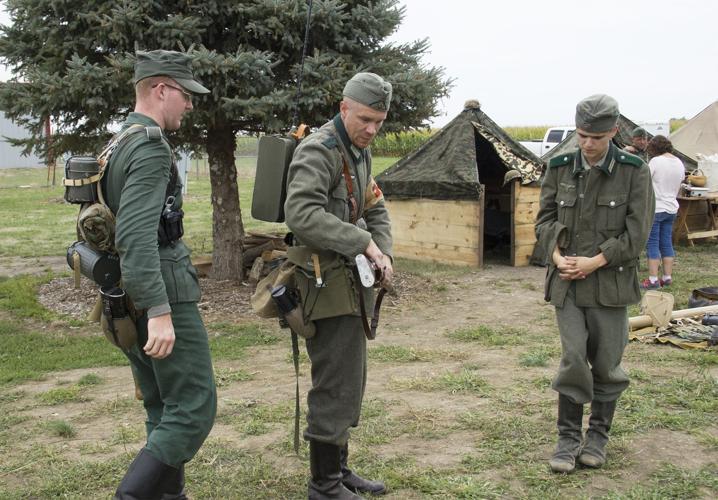This photograph depicts a group of three soldiers, seemingly engaged in a historical reenactment given the presence of modern-day elements like an individual in jeans and a t-shirt in the background. The soldiers are standing on a primarily dirt-covered area punctuated by sparse patches of grass. To the left in the background stands a tree, possibly a pine, adorned with green vines. There is also a small wooden hut with a black canopy.

The soldiers are dressed in a mix of dark and light green military uniforms, which appear to be from a past era, possibly the Civil War, and they all wear hats. The soldier on the left is in a dark green outfit, carrying various items on his back including a likely water canteen. The middle soldier, seen from his right side, wears a lighter green uniform and holds a gun, the butt of which is visible in his right hand, along with equipment strapped to his back and belt. The rightmost soldier, also in light green, is walking towards the viewer. These detailed uniforms include long sleeves, long pants, boots, bed palettes, and canteens, completing their historical appearance.